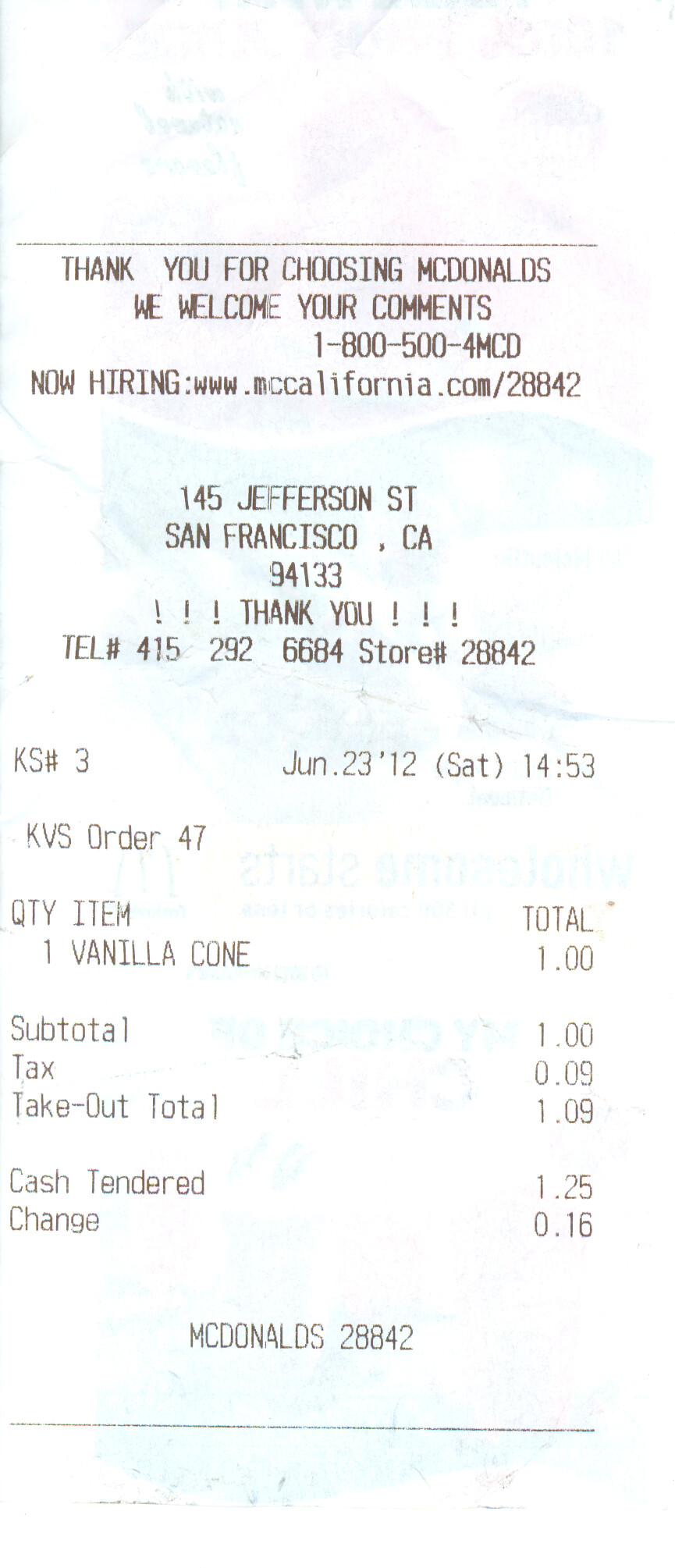The image features a receipt set against a completely white background, giving the impression that it could be a photocopy. Subtle imprints or ink bleeding through from the backside of the receipt introduce hints of green and red, though it is difficult to ascertain their exact source due to the photocopy effect.

The receipt is printed in black letters and begins with a message: "Thank you for choosing McDonald's." It invites customer feedback with the phone number "1-800-500-4MCD" and mentions job opportunities at "www.mccalifornia.com/28842." Below this, it lists the address "145 Jefferson Street, San Francisco, California 94113."

Further details provided include the store number "28842" and its contact telephone number "415-292-6684." The receipt is dated "June 23rd" and marked with an asterisk beside the number "12," indicating the hour when the purchase was made, which is "Saturday at 14:53." Additional specifics about the order are noted towards the bottom but are not entirely clear in the provided description.